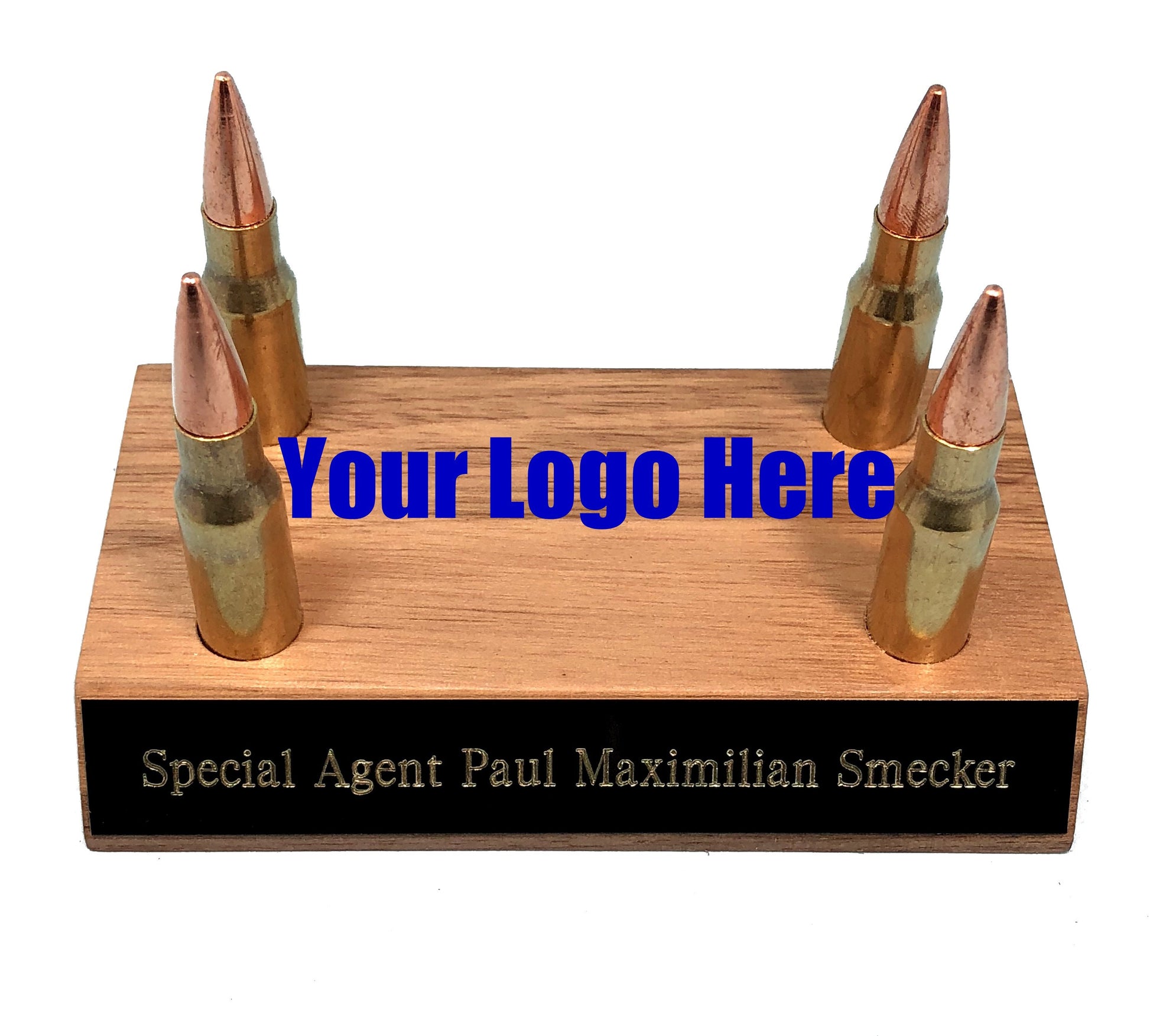The image depicts a promotional desk accessory that appears to be a combination of a nameplate and a paperweight. The central feature is a rectangular wooden block, approximately the size of a deck of cards, fashioned from light-colored wood. On the front edge of the block, there is a black nameplate with engraved white text that reads, "Special Agent Paul Maximilian Smecker." 

Mounted on the top surface of the wooden block are four large caliber bullets standing upright, two positioned on each corner. Between the sets of bullets, in blue block lettering that looks superimposed rather than engraved, the text "Your Logo Here" is prominently displayed, suggesting a customizable promotional product. The image is presented against a plain white background, emphasizing the item without any additional context or branding.